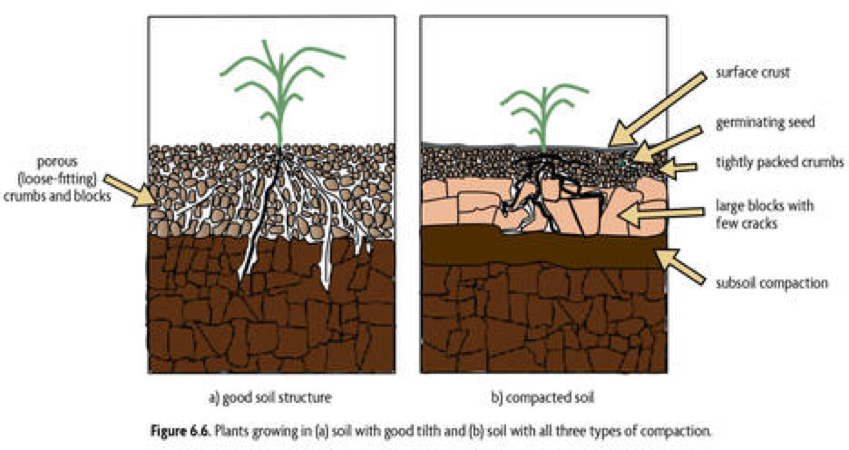This illustration is divided into two vertically aligned panels, each displaying a different type of soil structure with plants growing from them. The left panel (A) is labeled "good soil structure" and shows a green plant sprouting from the ground. This panel depicts a well-structured soil profile with distinct layers: the top layer has the plant with visible roots extending into a mid-layer of brown and grey circles (pebbles and blocks), followed by a bottom layer of uniform brown soil which the plant roots also penetrate. Adjacent to this diagram are terms like "porous (loose fitting)," "crumbs and blocks," with an arrow pointing to the mid-layer.

The right panel (B) is labeled "compacted soil" and features a smaller green plant sprouting from the ground. This diagram includes additional layers compared to the left. The top layer contains black pellets, labeled with arrows indicating "surface crust" and "germinating seed." Below this, a thin layer described as "tightly packed crumbs" sits above a distinct pink layer marked as "large blocks with few cracks." Further down, "subsoil compaction" is indicated just above a similar uniform brown bottom layer seen in the left panel. At the bottom of the image, it reads: "Figure 6.6. Plants growing in A) soil with good tilth and B) soil with all three types of compaction."